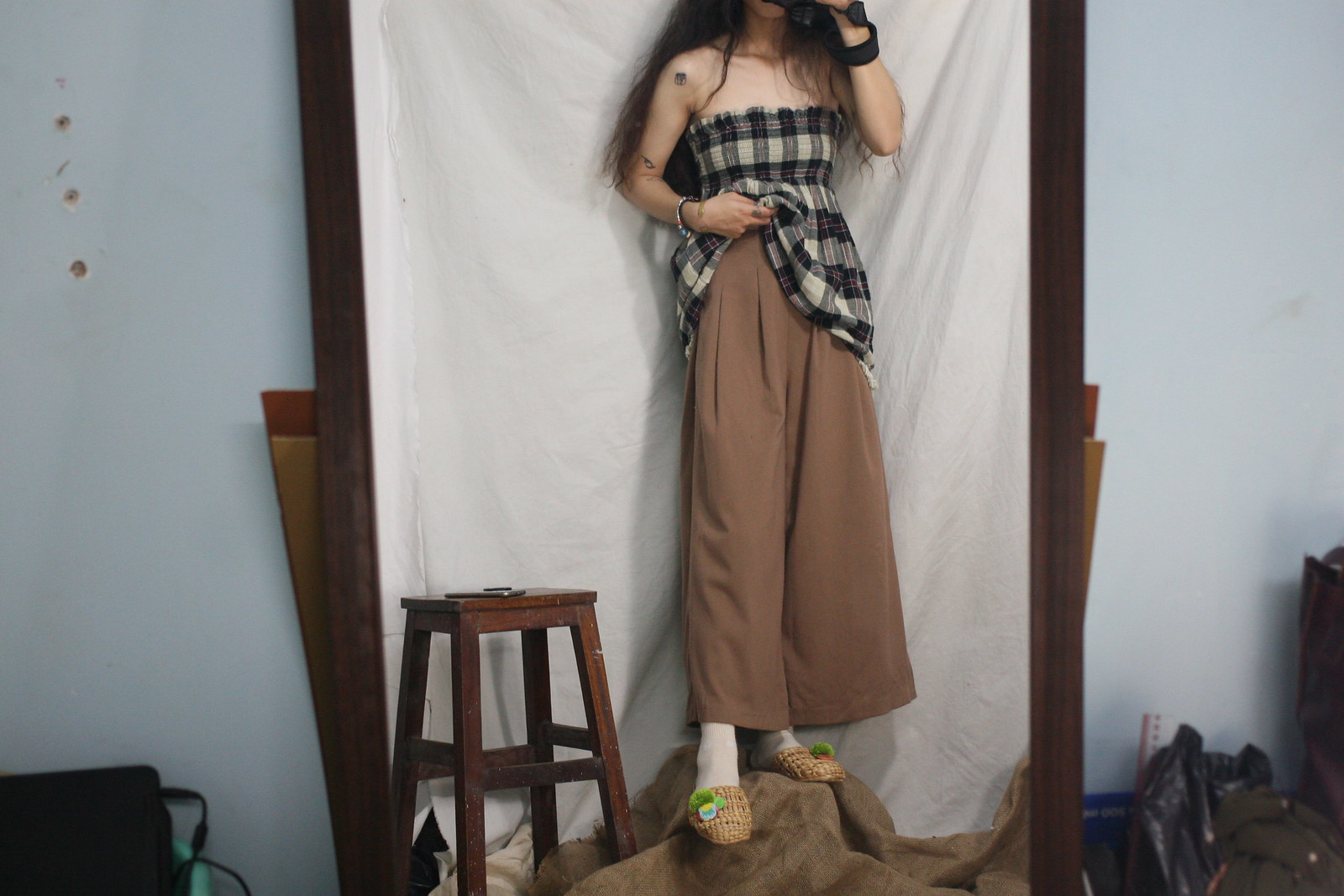In this photograph, a slender Caucasian woman is posed against a white backdrop. Her long, dark, slightly wavy hair cascades down her back, and she is dressed in a strapless black-and-white checked top with elastic, which drapes down to tunic length. With her right hand, she holds the top at her waist, revealing a bracelet on her wrist. She also has two small tattoos on her upper arm. She is outfitted in wide-legged, brown knit pants with two pleats at the top. Her feet are adorned with basket-like woven sandals, each decorated with a colorful cluster of pom poms, prominently featuring a bright green pom pom.

To her left, a dark brown wooden stool with a phone laying on it is visible. The woman stands on a burlap pile, which provides a textured contrast to the minimalist backdrop. The setting appears informal, and there is a hint of disorder in the room with damaged walls, marked by noticeable holes and clutter scattered about.